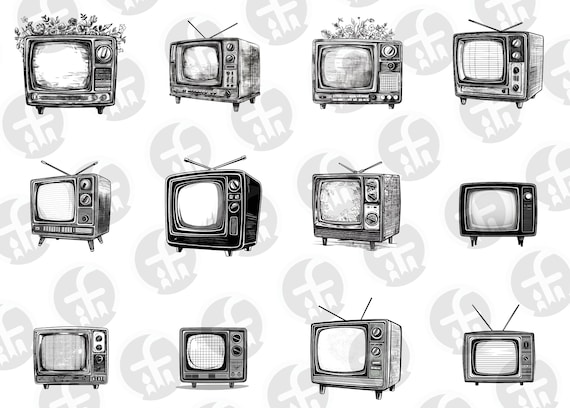The image showcases a grid of 12 pencil-sketch illustrations of vintage box-style televisions, arranged in three rows and four columns. The entire background is adorned with a repeating watermark that features a stylized lowercase letter "F" with a white candle beneath it and an unclear symbol on the right side of the "F," all set against a grayish backdrop.

Starting from the top left, the first TV is front-facing with flowers placed on top and stands on two legs. To its immediate right is a television with a two-prong antenna, positioned diagonally, showing three of its feet. The third TV also has flowers on top and stands on two visible legs. The fourth in the top row is another antenna-equipped set.

In the second row, on the far left, is a three-legged TV with bunny ear antennas. To its right, there is a slightly larger, darker television with an antenna. The third TV in the second row also has a two-prong antenna and is darker than the first but lighter than the second. The last in this row is a smaller, almost completely black outline TV.

The bottom row begins with a medium-shaded television without antennas or flowers. Next to it is a slightly narrower TV with no decorations, facing forward. Following this is a diagonal-facing TV equipped with two dials, a two-prong antenna, and three visible feet. The final television in the bottom row is one of the smaller sets, featuring a two-prong antenna and two visible feet, with unclear knob details.

All the televisions are distinctly drawn in black and white, embodying different nostalgic designs from the 1960s and 70s, with half adorned with traditional bunny-ear antennas and others lacking any external fixtures.